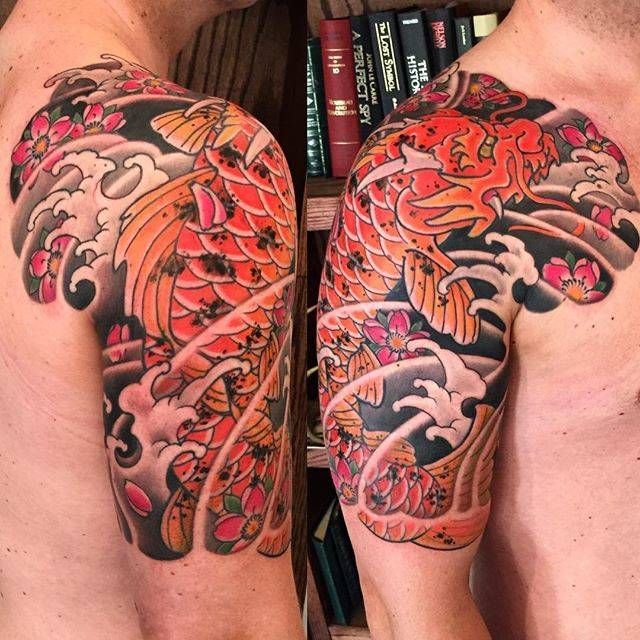This image features two side-by-side photos of a vibrant Japanese traditional-style tattoo on a white male. The left photo displays the back view, while the right photo reveals the front view, including parts of the chest. The tattoo, rich in colors like orange, pink, black, white, and gray, spans from the base of the neckline down to nearly the elbow, wrapping halfway down the shoulder blade and the bicep. The central design is an ornate orange koi fish with a dragon head, featuring one visible fang and a gold eye, along with black specks on its body resembling dog prints. Complementing the koi are intricate black and white waves and water lines, along with several pink lotus flowers and white orchids, one notably near the armpit.